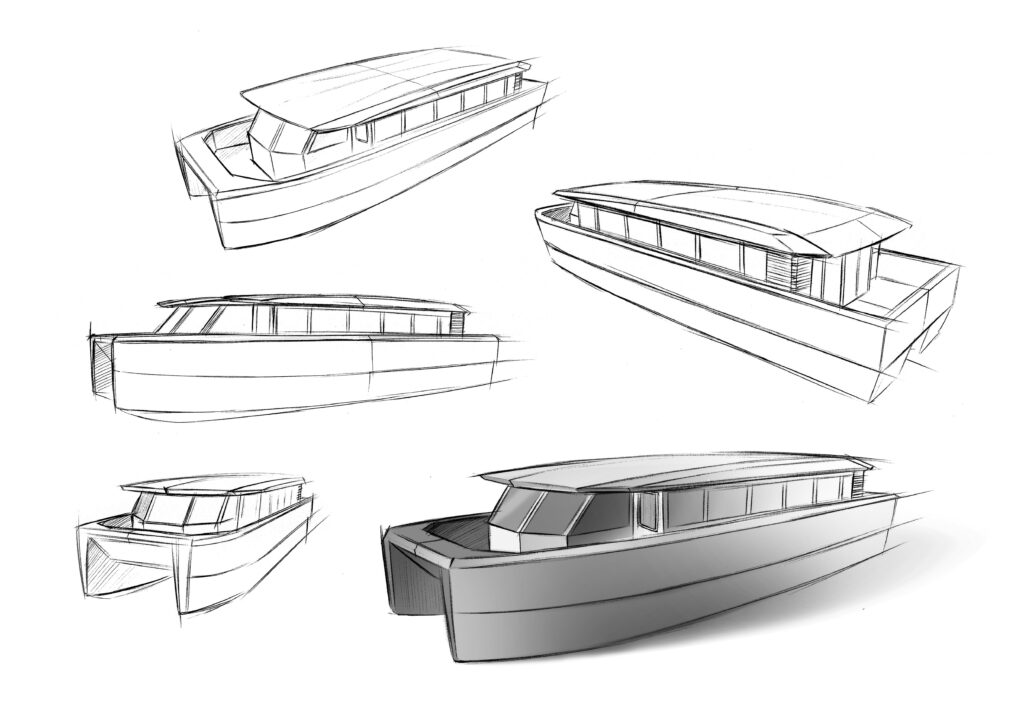The image features five detailed sketches of a boat against a white background. Each sketch represents a different perspective and stage of the boat's design process. The sketch at the bottom right is the most detailed, shaded in gray, showcasing the boat's full form. To the left of this, moving upwards, are three more sketches rendered in black pencil. The bottom left sketch provides a front view, the next one up depicts the left side, and the topmost sketch is a top-down view. Lastly, the rightmost sketch shows another view from the left. The boat design features a lower and upper deck, numerous glass windows, a roof, and a wooden outer border, seen across the various stages of the drawing.